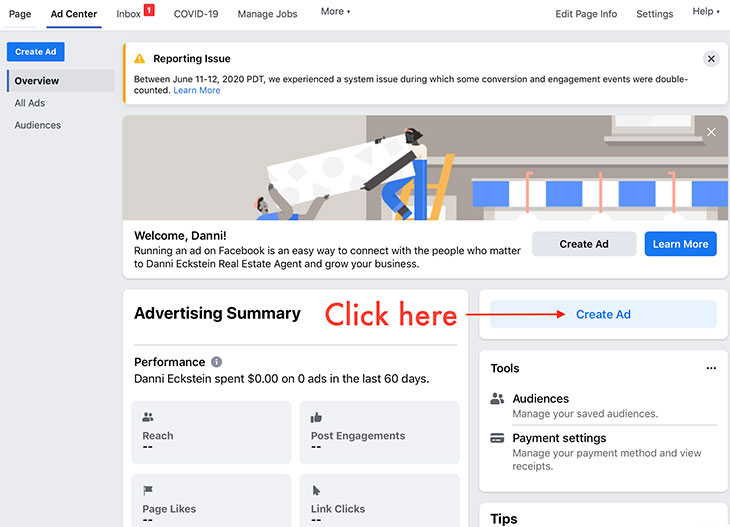"Screenshot of the Facebook Ad Center Dashboard:

At the very top, the page title 'Page Ad Center' is displayed in bold black text on a white background, and it is underlined for emphasis. Directly below, there is an inbox notification with a red square and the number '1' inside it. The text 'COVID-19 Managed Jobs' is listed next, followed by the option 'More.'

On the far left, a blue box prominently labeled 'Create Ad' is visible. Beneath it, a navigation menu includes options such as 'Overview,' 'All Ads,' and 'Audiences.' Moving to the right, the next column features a notice titled 'Reporting Issue' next to a yellow triangle. The notice reads: 'Between June 11th and 12th, 2020, we experienced a system issue during which some conversion and engagement events were double counted. Learn more,' with the 'Learn more' text highlighted in blue.

Below the notice, there is an illustration of a man and a girl putting up an awning in front of a building. The girl stands on a ladder while the man assists her from the ground. Underneath the image, text reads: 'Welcome Dan, running an ad on Facebook is an easy way to connect with people who matter to Danny Eksterstein, the real estate agent, and grow your business.' To the right of this text, there are two clickable buttons: a gray 'Create Ad' button and a blue 'Learn More' button.

Further down, the section is labeled 'Advertising Summary.' In large, red letters that draw immediate attention, it says 'Click here,' with an arrow pointing directly to another 'Create Ad' button in a blue box.

Overall, the screenshot captures various elements of the Facebook Ad Center interface designed to guide users in creating and managing advertisements, while also addressing a recent system issue."